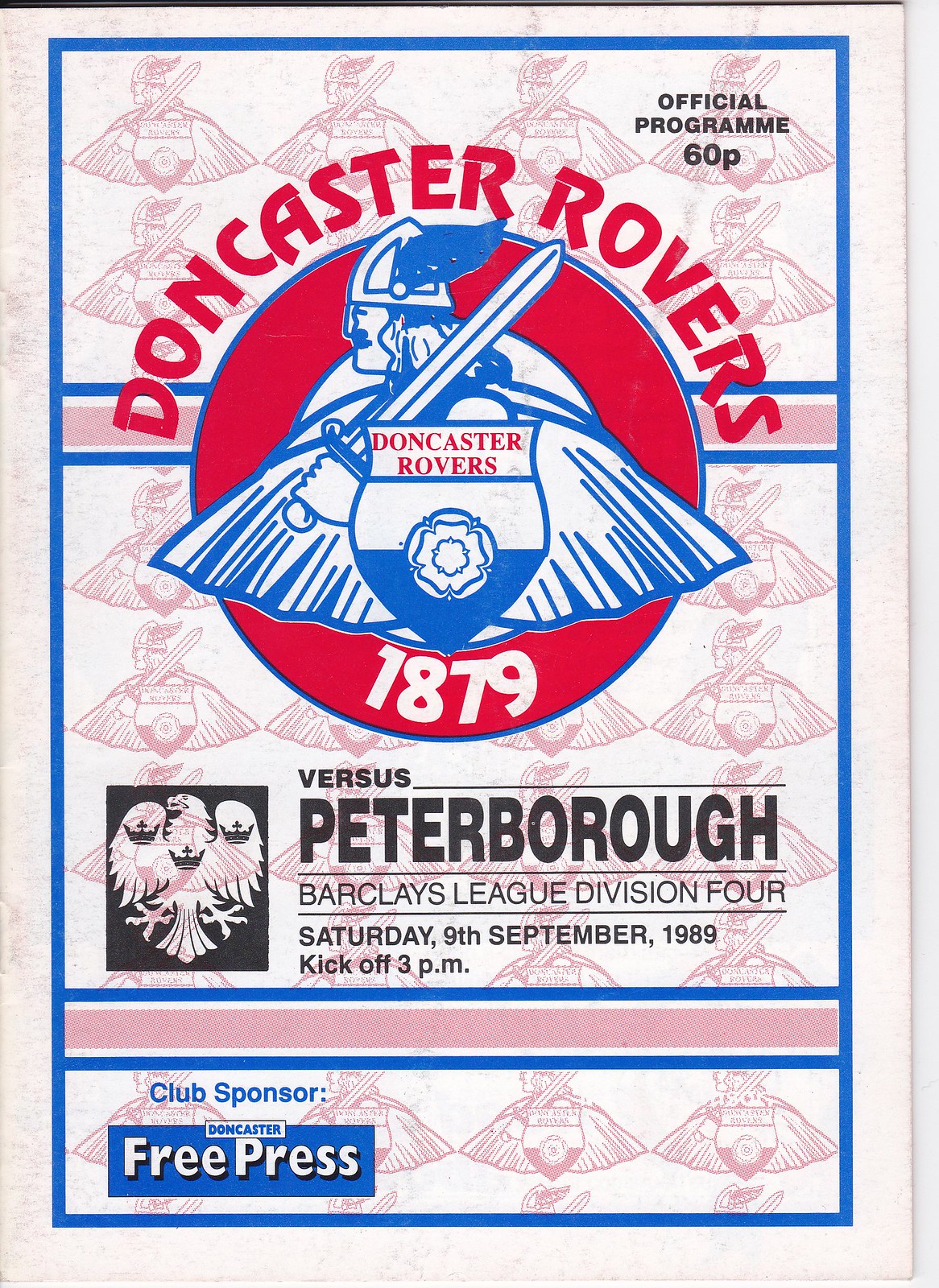This is a detailed caption of an image of a vintage Doncaster Rovers football poster:

The central feature of the poster is the Doncaster Rovers logo, which prominently displays a man carrying a sword. Surrounding this figure is a red circle, within which "Doncaster Rovers" is prominently written. Directly below this circle, the founding year "1879" is inscribed, and again, the words "Doncaster Rovers" are arching over the top of the circle. 

In the top right corner of the poster, the text "Official Program 60P" is visible. Beneath the central logo, text announces a matchup: "Versus Peterborough Barclays League Division Four, Saturday 9th September 1989, Kickoff 3 p.m." 

To the left of the central logo, there's a black and white logo resembling an eagle. Beneath the eagle logo lies a pink horizontal strip with the text "Club Sponsor Free Press" inscribed on it. 

The poster is bordered by a blue line. Its background features a light pink color adorned with a repeated, slightly transparent replica of the central Doncaster Rovers logo.